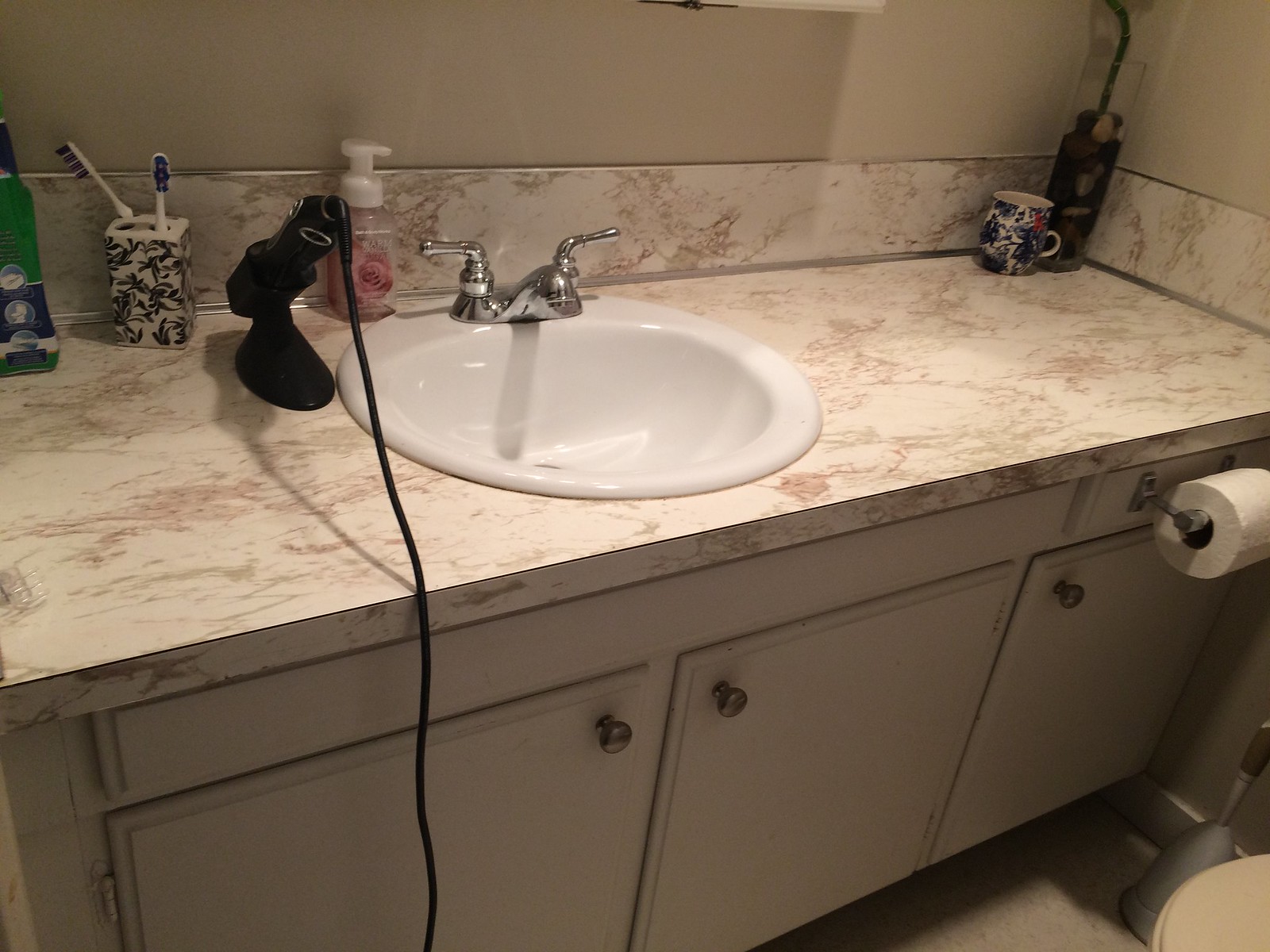This photo captures a detailed view of a bathroom countertop, showcasing its luxurious white marble surface adorned with subtle pink veining. At the center of the countertop is a pristine white sink, complemented by a sleek, silver faucet set, with separate hot and cold handles. 

To the right, a chic pump bottle of soap features a delicate pink rose design and white lettering on the top, adding a touch of floral elegance. To the left, a hair styling tool, possibly a curler or straightener, is neatly stored in a designated holder with a visible cord trailing down. Adjacent to this is a white toothbrush holder, adorned with blue floral patterns, containing two manual toothbrushes in separate slots.

Further left, a bottle of mouthwash is stationed, ensuring dental hygiene essentials are within reach. On the far right side of the countertop, a matching floral mug echoes the design of the toothbrush holder, adding a cohesive decorative touch.

Below the countertop, a wooden vanity features a long central drawer and two cupboard doors with small knobs. To the right of these, another cupboard is visible. The beige walls are partially adorned with a white-framed mirror with gold detailing, subtly reflected at the top of the image.

Additionally, mounted to the side of the cabinet is a silver toilet paper holder, with a roll of toilet paper extending from it. On the floor below, a toilet plunger and part of the toilet itself are visible, completing the practical aspects of the bathroom setup.